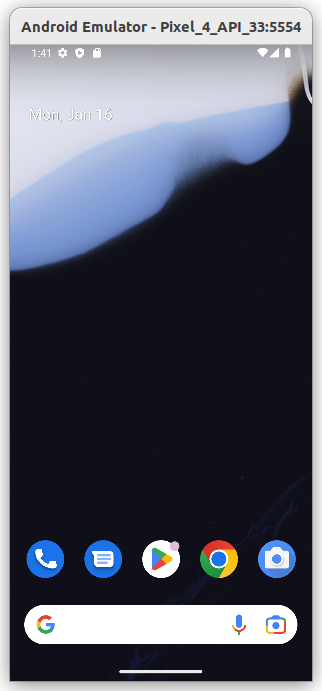This image depicts an Android emulator running on a PC. At the top, the emulator is labeled as "Pixel_4_API_33:5554." The emulator screen showcases the Android home page, adorned with a heavily accentuated drop shadow around the edges, adding a somewhat exaggerated visual effect.

The status bar at the top displays the time "1:41," along with typical icons such as a gear icon for settings, a badge with a play button, a shopping cart, Wi-Fi signal, and battery strength indicators.

The background image is primarily light gray, featuring an angular splash of light blue at the upper left and a gradient of darker blue to black rising from the bottom. The lower right corner includes small graphic elements resembling pebbles or miniature rocks, contributing to a more artistic rather than photographic look.

The upper left corner indicates the date as "Monday, January 16th." Along the bottom of the screen, there are five essential app icons for Phone, Chat, Play Store, Chrome, and Camera. Below these, the search field is prominently placed, featuring a "G" logo on the left and microphone and camera icons on the right, facilitating voice or image search options.

Overall, this well-detailed emulator display provides an immersive Android experience on a PC.